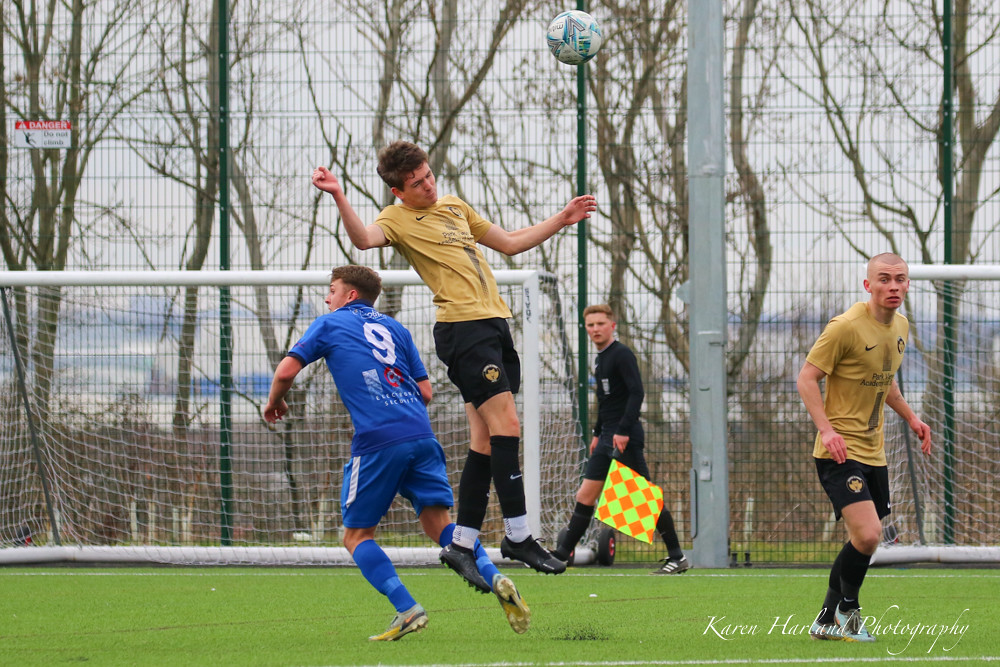The image captures an outdoor soccer game between two teams, one wearing gold and black and the other in all blue. Central to the action, a player from the gold and black team is mid-air, heading the ball towards his teammates. The player wears black shorts, black socks, and black shoes. His opponent from the blue team is also in the shot, challenging for the ball. In the background stands a referee or linesman, dressed in black and holding a lime green and orange checkered flag, attentively watching the play. The field is lush green, suggesting it might be springtime, despite the leafless trees in the distance. Behind the players, two soccer goals are visible, with a net and a large steel pole supporting a chain link fence featuring a "Danger: Do Not Climb" sign. The overcast sky adds to the scene's dynamic atmosphere.